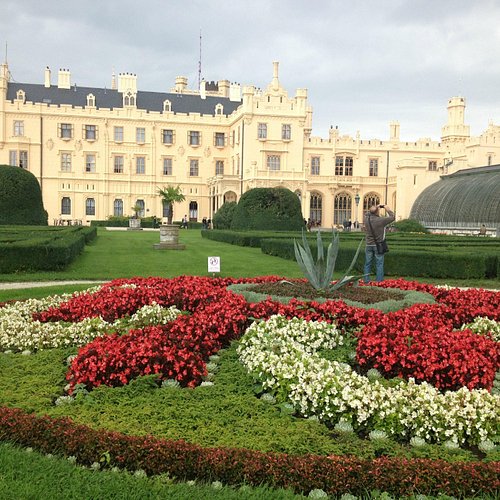The image depicts a grand palatial structure that could be a historic government building, royal institution, or even a lavish hotel. The architecture features an ornate design with cream and yellow-colored walls, and a charcoal gray roof. This three-story edifice boasts large windows with multiple panes, with the ground floor particularly highlighted by enormous arching windows. 

In the foreground, there is an exquisitely manicured garden with circular flower arrangements in red and white, intricate hedges, and cement flower pots. A significant cement fountain, cascading water dramatically, serves as a central focal point amidst the lush greenery. Additionally, a gentleman tourist is captured pointing his camera or cell phone toward the majestic building, adding a human element to the serene landscape. The sky above is overcast and cloudy, casting soft shadows over the picturesque scene.